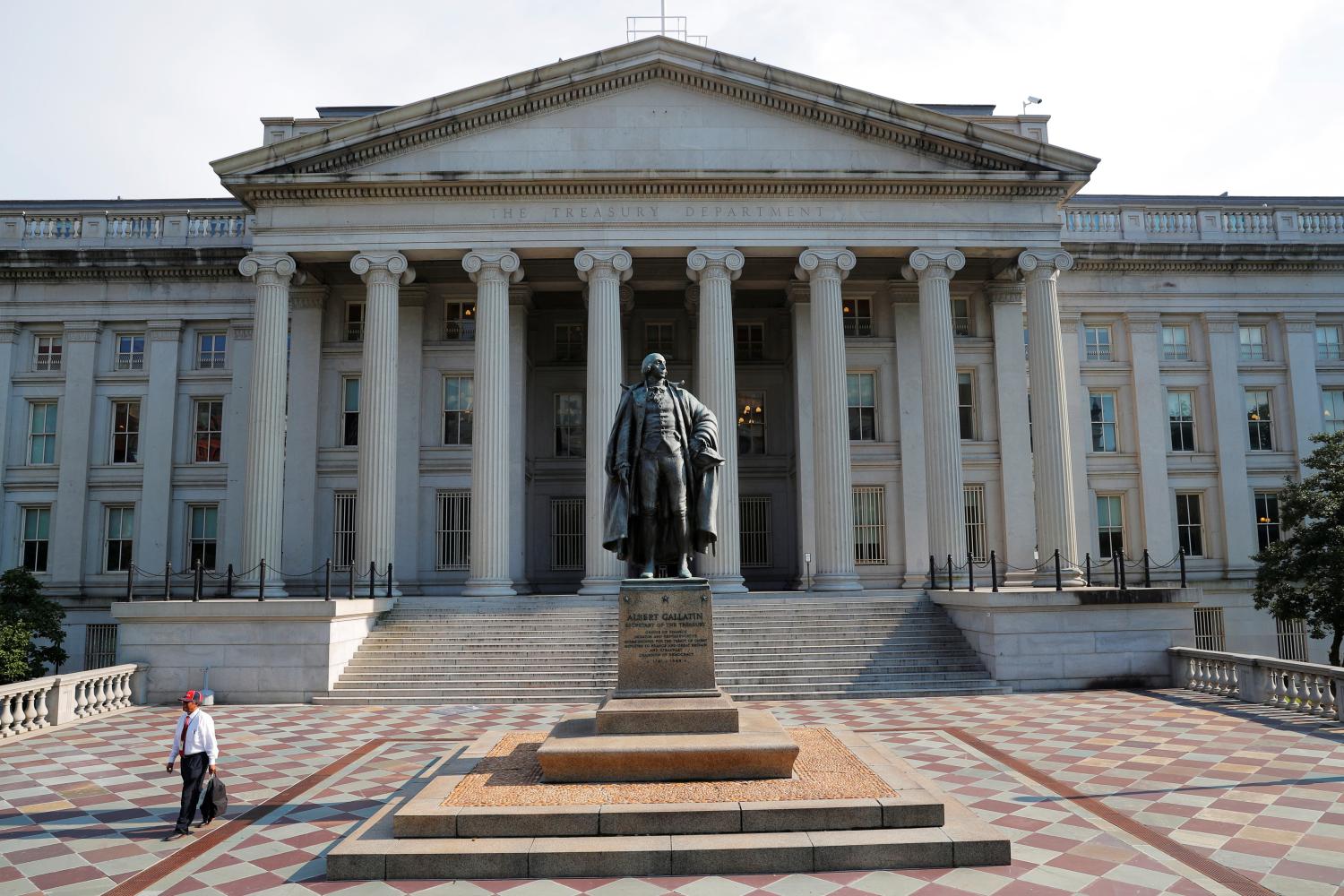This color photograph, in landscape orientation, resembles a picture postcard and captures a majestic, Roman-style U.S. Treasury Department building under a clear, sunny sky. The imposing stone structure features a large peaked roof supported by a grand array of eight carved columns that form a portico. Below the roof, bold engravings affirm the building’s identity as the Treasury Department. Leading to this entrance is a broad, low staircase composed of approximately 15 to 20 steps.

In front of this impressive building lies a plaza adorned with a distinctive, diagonal checkerboard pattern of red and gray pavers. Dominating the plaza is a bronze statue on a pedestal, portraying a man in colonial attire, complete with a long coat, vest, pants, boots, and a colonial wig. This stately figure stands with one hand on his hip, gazing skyward, exuding an air of pride and historical significance. Although the inscription on the statue is unreadable, hinting it might not be George Washington, the figure's attire suggests a prominent historical persona from the 1700s.

The scene is brought to life by the presence of a lone man, potentially a tourist or a worker, distinguishable by his red baseball cap, white long-sleeved shirt, dress pants, and a backpack in his left hand. He walks away from the statue, adding a sense of scale and movement to the otherwise timeless and serene setting. Lush trees frame either side of the grand building, completing this harmonious and picturesque composition.